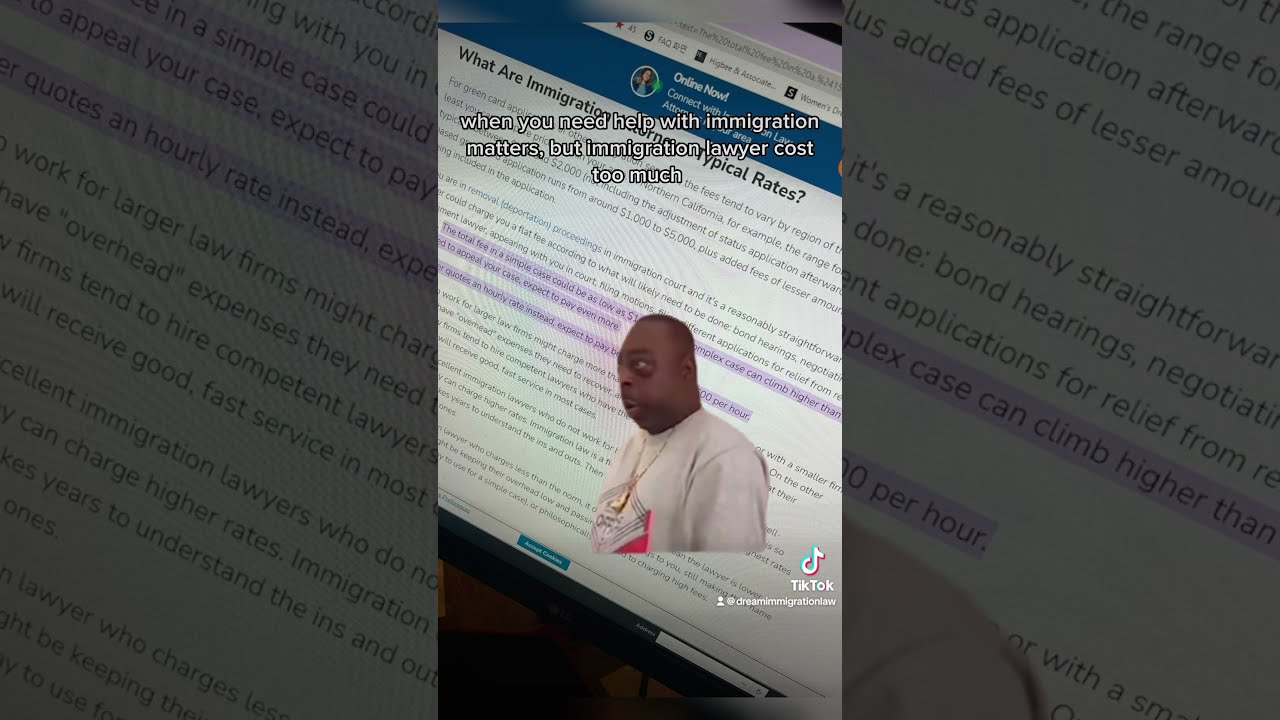The image is a screenshot of a TikTok video featuring a meme about the high costs of immigration lawyers. The TikTok watermark is present, reading "TikTok at Dreaming Immigration Law," with the recognizable TikTok logo in the bottom right corner. The screenshot is taken at an angle so the top of the website is towards the top right corner and the bottom is towards the top left corner. Overlaid text in white at the top center reads, "when you need help with immigration matters, the immigration lawyer costs too much," though there's a noted grammar error. In the foreground, a black man is visible from the chest upwards, turned to the left. He's wearing a white shirt with a black wrestling ring graphic and a gold chain around his neck. His expression appears surprised, with wide-open eyes and a slightly open mouth. Some of the website’s text beneath him reads, "what are immigration attorneys' typical rates," with parts highlighted in purple.